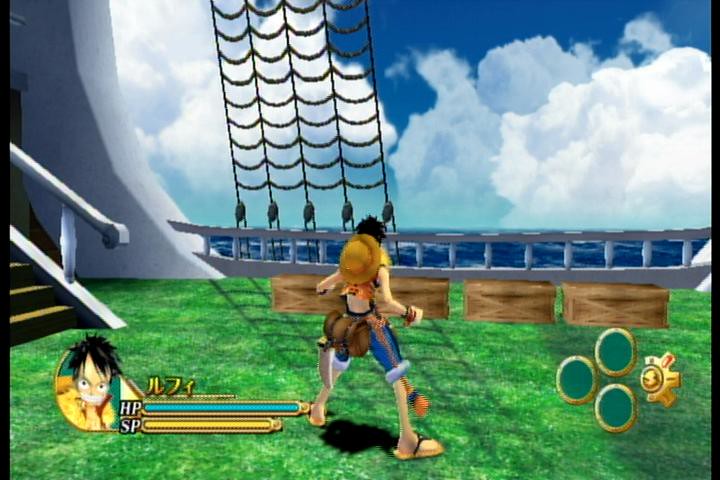In this detailed drawing, we observe a scene that seems to be captured from a ship or a platform adjacent to a large body of water. The background is dominated by an expansive water view, accompanied by clouds that fill the sky. On the left side of the composition, a series of ropes extend upward and appear to be tied to a railing visible in the background. Additionally, a staircase—which is unusual for a typical ship setting—suggests that this might be a platform located near the water.

In the foreground, there is an exaggerated caricature of a person gazing out toward the open water. This individual is adorned with a pith helmet that hangs across their back by a strap over their shoulders, rather than being worn on their head. The character exudes a fighter's aura, with a belt potentially for a knife slung on their left side and sandals on their feet. Their dark hair and the intense posture, with hands clenched and arms bent and extended outwards, add to their resolute appearance.

At the bottom of the drawing, indicators resembling those from a game interface are present. One label reads "HP" with a long blue line next to it, while another label reads "SP" with a shorter orange line. These suggest health points and possibly a special power or stamina meter, indicating that the artwork might be derived from a game. The character stands on a green surface that looks like either grass or a carpet designed to imitate grass, adding an additional layer of texture to the scene.